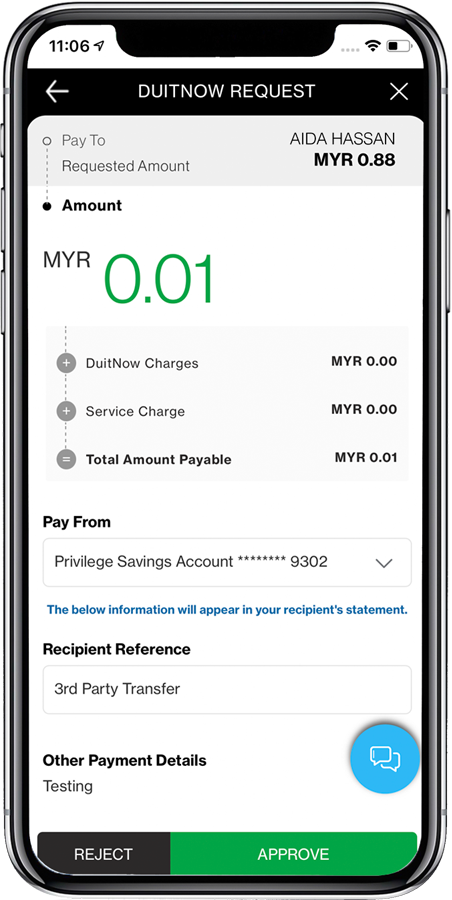Photograph of a smartphone screen displaying a payment request interface. The screen is in a vertical orientation and features a predominantly white background with subtle variations in light shading. The main elements of the interface are primarily in black text with bold highlights and include minor accents of green and blue.

At the top, there is a label "Do It Now Request" in white lettering against a black background. Directly below, a tab reads "Pay to requested amount" followed by the recipient's name, Ada Hassan, and the amount "MYR 0.88" in bold black text.

Further down, the screen displays an "Amount" section, highlighted with a bullet point and the term "MYR" (Malaysian Ringgit) in capital letters. The amount "0.01" is prominently shown in large green numbers.

The interface also provides detailed information on the app's charges, including "Do It Now Charges," "Service Charges," and the "Total Amount Payable," ultimately showing an amount of one penny. Below this, there's a section "Pay from," indicating that the payment will be made using the user's savings account, with the last four digits of the account number displayed in blue text.

At the bottom of the screen, a notice mentions that the below information will appear in the recipient's statement. The interface concludes with two action buttons: "Reject" in black on a white background and "Approve" in white on a green background.